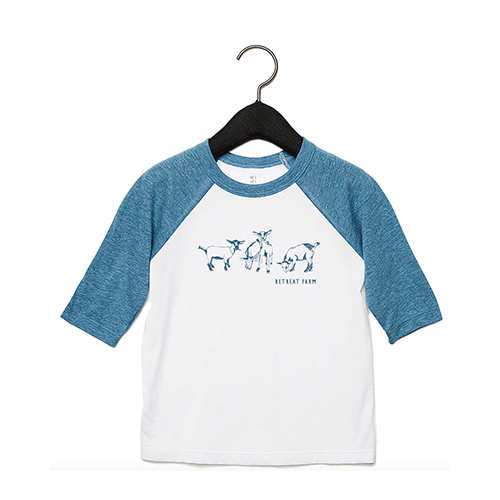This photograph features a child's t-shirt displayed on a black hanger with a silver metallic hook, set against an entirely white background, suggesting it could be used for online retail purposes. The t-shirt showcases a vivid color scheme with blue sleeves that extend up to the collar, which is also blue, while the main body of the shirt is white. Central to the design is an illustration of four goats, drawn in shades of blue and white to match the shirt's colors. Below the goat illustration, there is text that appears to read something akin to "Nettrent Farm" or similar, reinforcing a farm theme. The lower portion of the shirt is left plain white, enhancing its simplicity and drawing attention to the central design. Judging by its size and design, the shirt is specifically tailored for children.